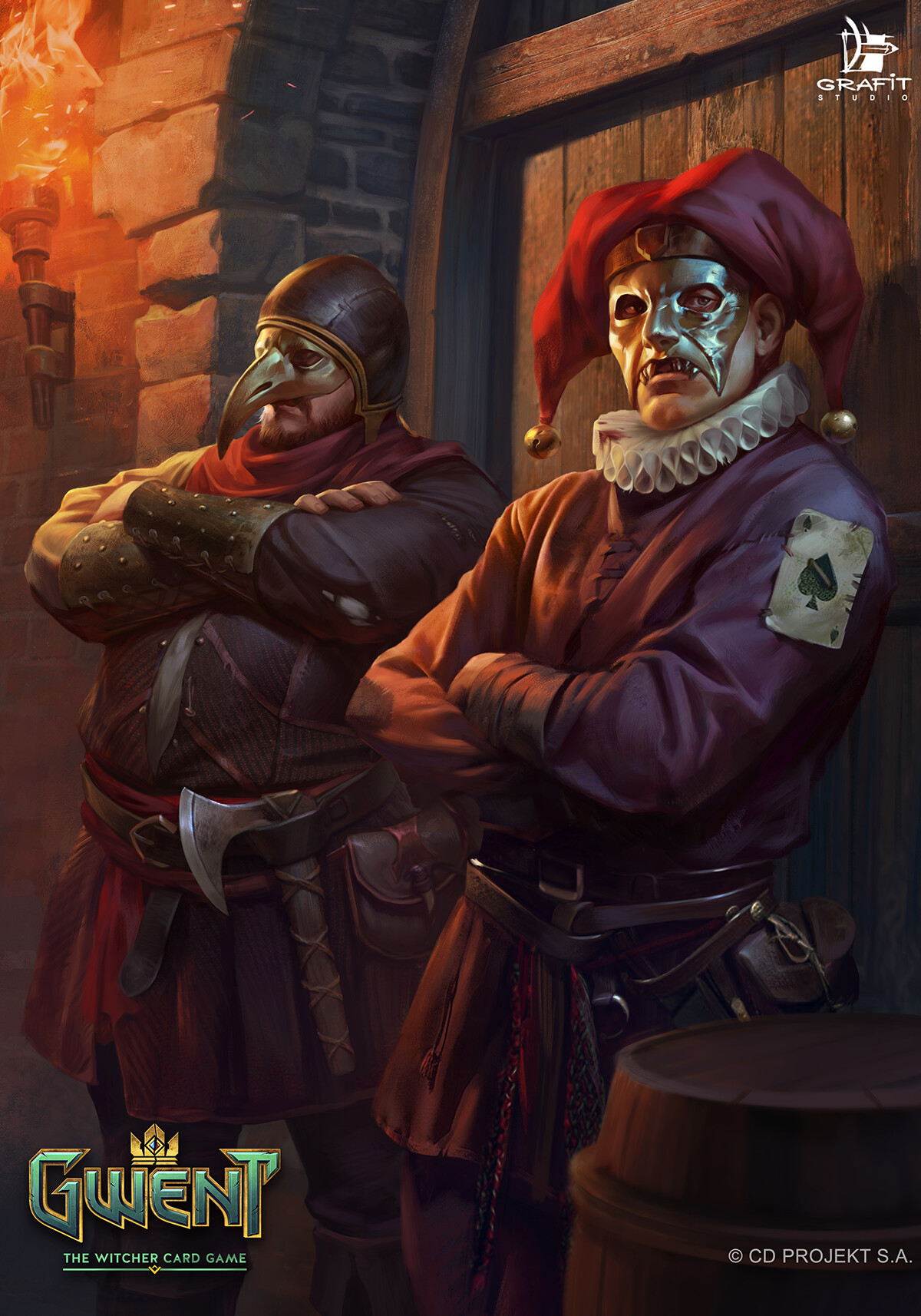In this detailed image from the computer game "GWENT: The Witcher Card Game," we observe two distinctive men standing guard in what appears to be a torch-lit dungeon or stone room. On the left, a stout man is clad in a brown jersey with a red portion extending to the floor, complemented by a red-brown scarf around his neck. His appearance is notable for a gray metallic helmet with a silver mask covering his eyes and ending in a prominent beak, reminiscent of a plague doctor. Leather arm protectors cover his wrists, and a large hatchet hangs from a leather belt around his waist. His hands are crossed in front of him as he leans against a wooden door made of dark vertical wooden slats.

To his right stands a man dressed as a jester, donning a vibrant red hat with tassels ending in bells and a mask that resembles an ogre with elongated teeth. His outfit is a mix of purple, brown, and reddish hues, including a patch with a spade on his left bicep. He wears a ruffled white collar around his neck and a belt that holds a leather pouch. A wooden barrel with vertical slats is positioned in the lower right corner, adding to the scene's medieval ambiance. Together, these two characters appear to be vigilantly guarding whatever lies behind the imposing wooden door.